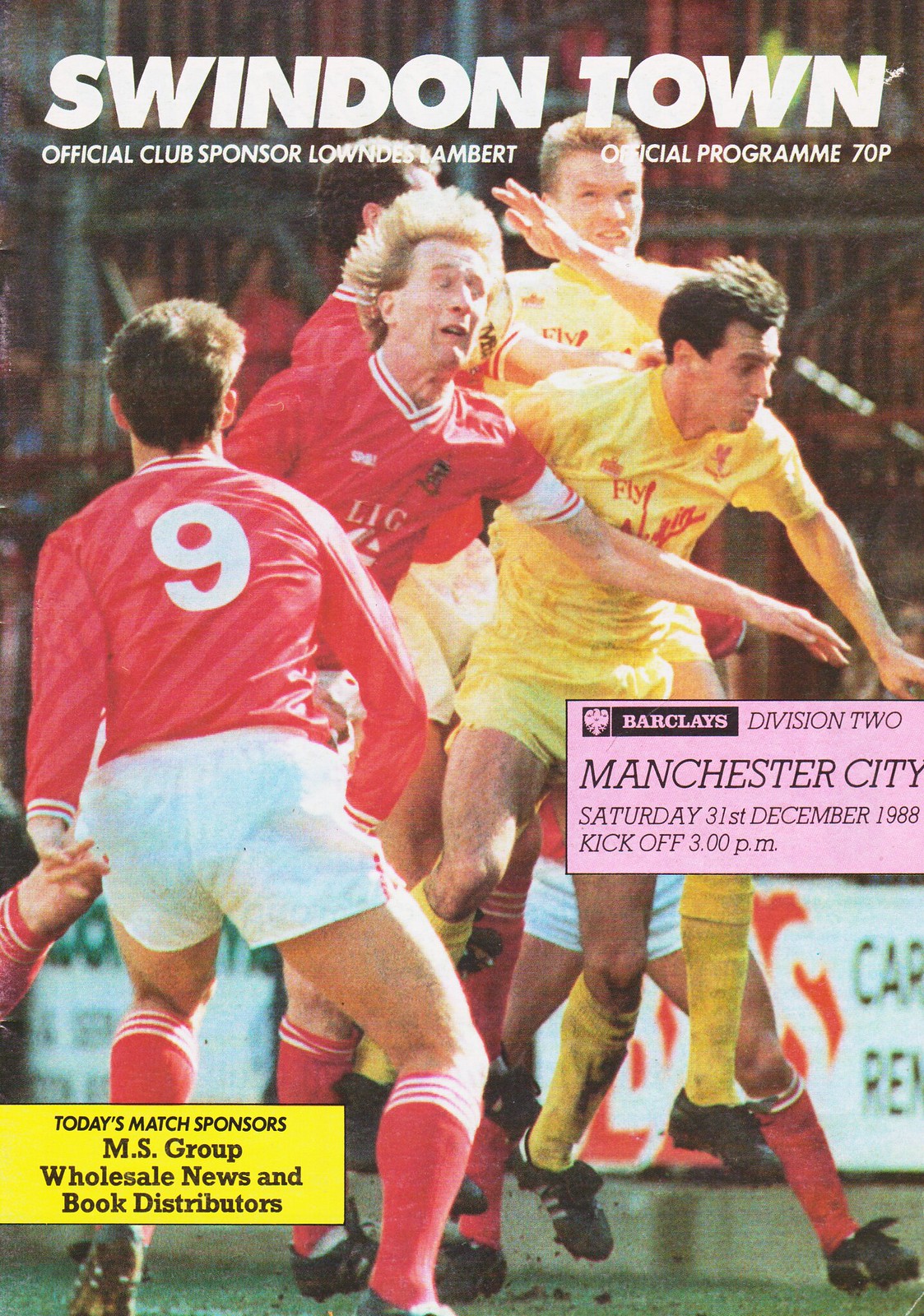The front cover of the European football (soccer) league program features a dynamic action shot of a match between Swindon Town and Manchester City, dated Saturday, 31st December 1988, with a 3 p.m. kickoff. Priced at 70p, the program highlights the official club sponsor, Loudon's Amber. The cover showcases a vivid scene with five players: three clad in red jerseys and white shorts, representing Swindon Town, and two in all-yellow uniforms with red text, representing Manchester City. The players are intensely engaged in the game, with two players leaping into the air, likely contesting a header, while others are running, blocking, and jostling each other. The text also includes mentions of today's match sponsors, CMS Group, Wholesale News, and Book Distributors. The number nine player, prominent and closest to the camera, further adds to the cover’s vibrancy and action-packed feel.